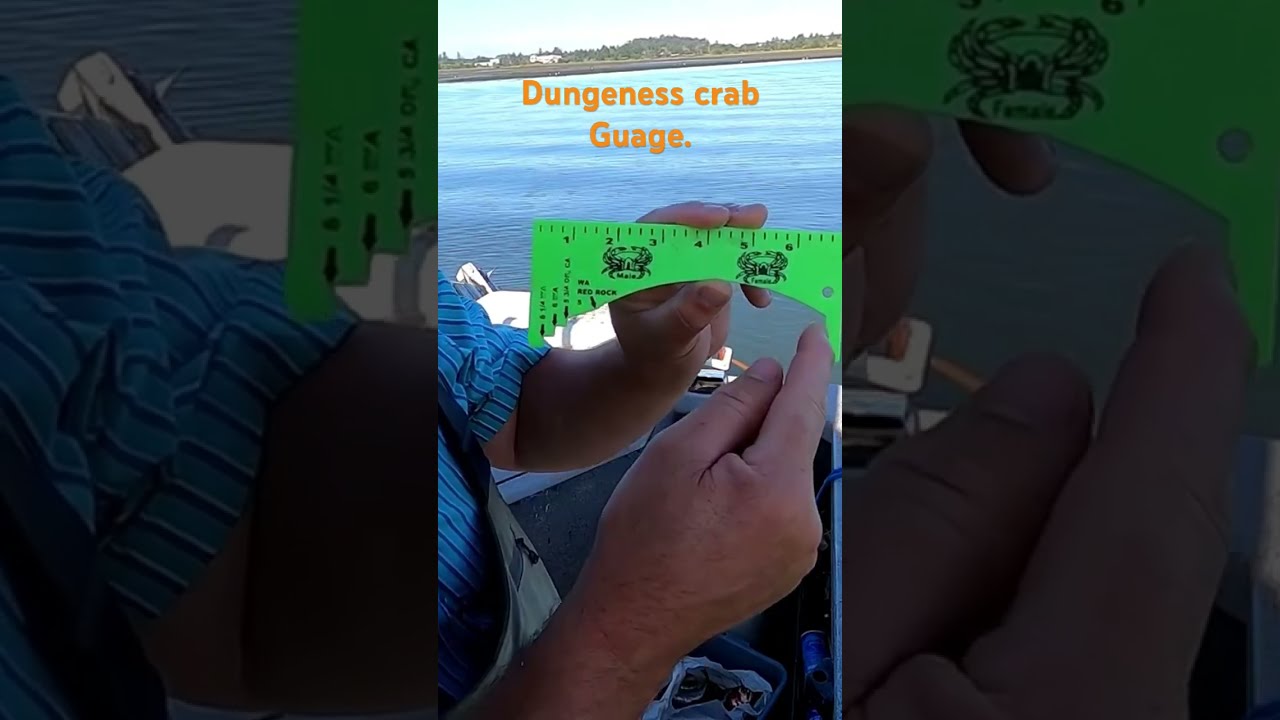The image features a horizontally rectangular, full-color photograph set in the middle, surrounded by a darkened close-up of the same photograph, creating a three-panel effect. The scene takes place outdoors during the daytime, on a calm blue body of water, possibly a river or lake, with a distant shoreline visible that has greenery and a blue sky above. In the central photograph, a white Caucasian male is aboard a boat. He is wearing a blue-striped shirt, and the visible parts of his body include his hands and arms, which have some hair. He is holding and pointing to a green measuring tool known as a "Dungeness Crab Gauge," used to determine whether crabs are of a keepable size. The gauge displays numerical markings from 1 to 6 inches, with lines in between for precision, and features an image of a crab. Overlaying the photograph, in orange text, are the words "Dungeness Crab Gauge."